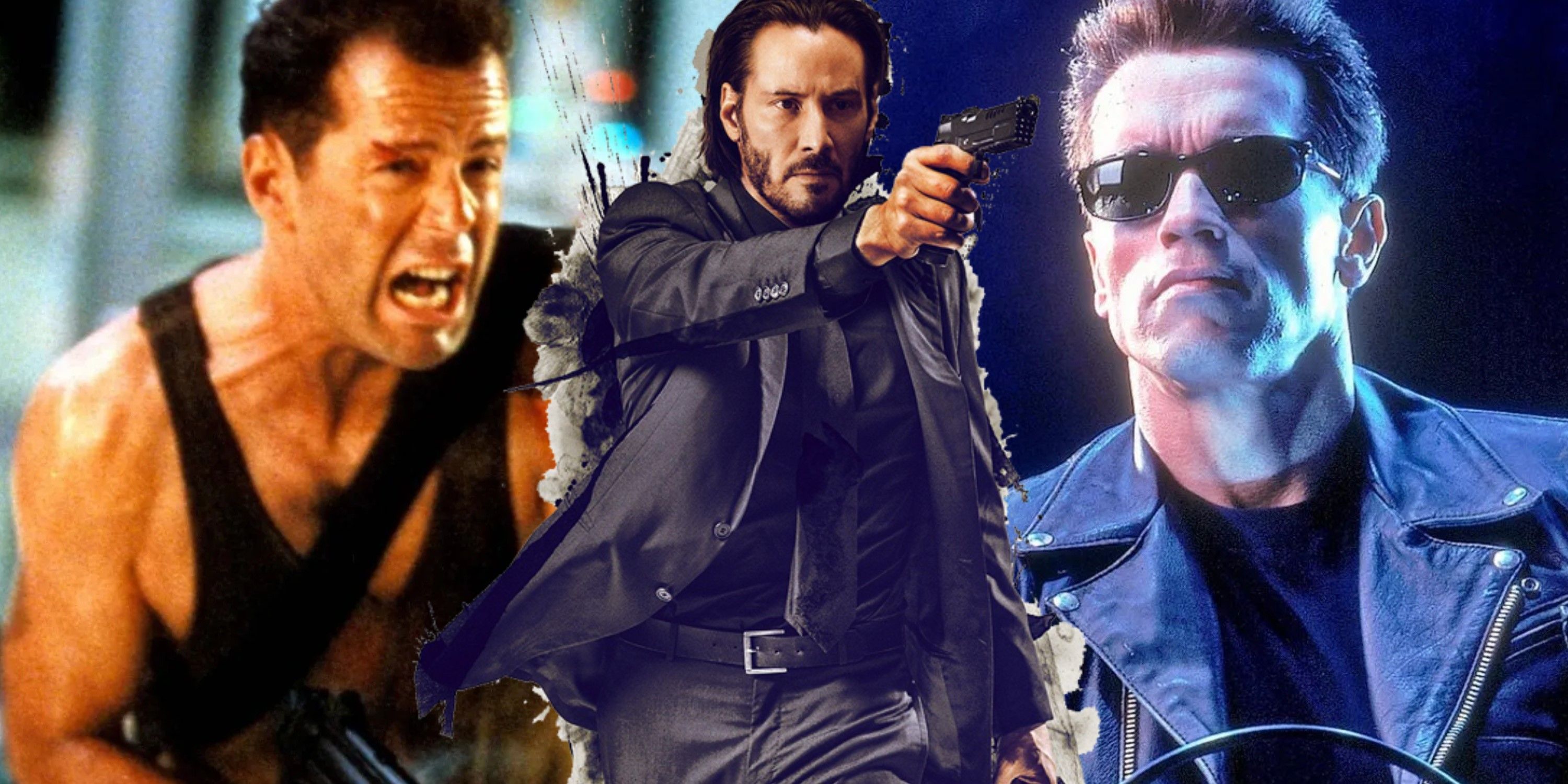The image features three iconic action movie actors, each from different films. On the left is a youthful Bruce Willis, recognizable from his "Die Hard" days, with dark hair, a shiny, muscular bare chest, and a black strap around his shoulders suggestive of a gun holster. He is making a determined face. In the center stands Keanu Reeves, dressed in a sleek black suit with a black shirt, tie, and pants, embodying his "John Wick" role. He has a black mustache and beard, holding a pistol in a shooting stance, and behind him is a torn, tattered backdrop. On the right is a young Arnold Schwarzenegger, from the "Terminator" series, with spiked brown hair, black sunglasses, a black t-shirt, and a black leather jacket. He appears to be riding a motorcycle against a dark, undefined background. Together, they represent three eras of classic action cinema.